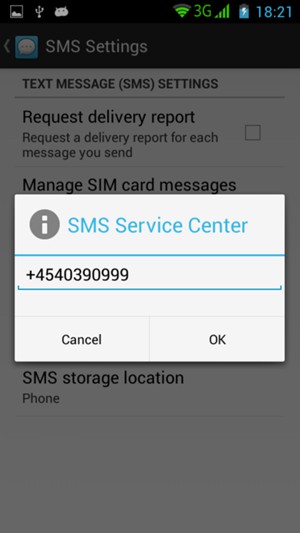A smartphone screenshot displays a detailed interface showcasing various information and settings. At the top, the status bar indicates a strong connectivity with 3 out of 4 Wi-Fi signal bars and full cellular reception with 4 bars, connected to a 3G network. The time is shown as 18:21 in blue text. 

Below the status bar, a blue notification box with a white text bubble containing 3 dots appears, suggesting ongoing messaging activity. The main display is predominantly black with areas highlighted in white. The black background features white uppercase text that reads "SMS Settings."

Beneath this title, on a white background, there is a prominent horizontal line followed by large, bold black text stating "Request Delivery Report." Directly underneath, in smaller font, the description "Request a delivery report for each message you send" is provided. To the right of this descriptive text, there is an unchecked checkbox.

Further down, another setting labeled "Manage SIM Card Messages" is noted. Upon interacting with this option, a white pop-up box titled "SMS Service Center" appears in blue text. Below, there is a black text displaying the service center number "+4540390999." At the bottom of this pop-up, there are two buttons: "Cancel" on the left and "OK" on the right.